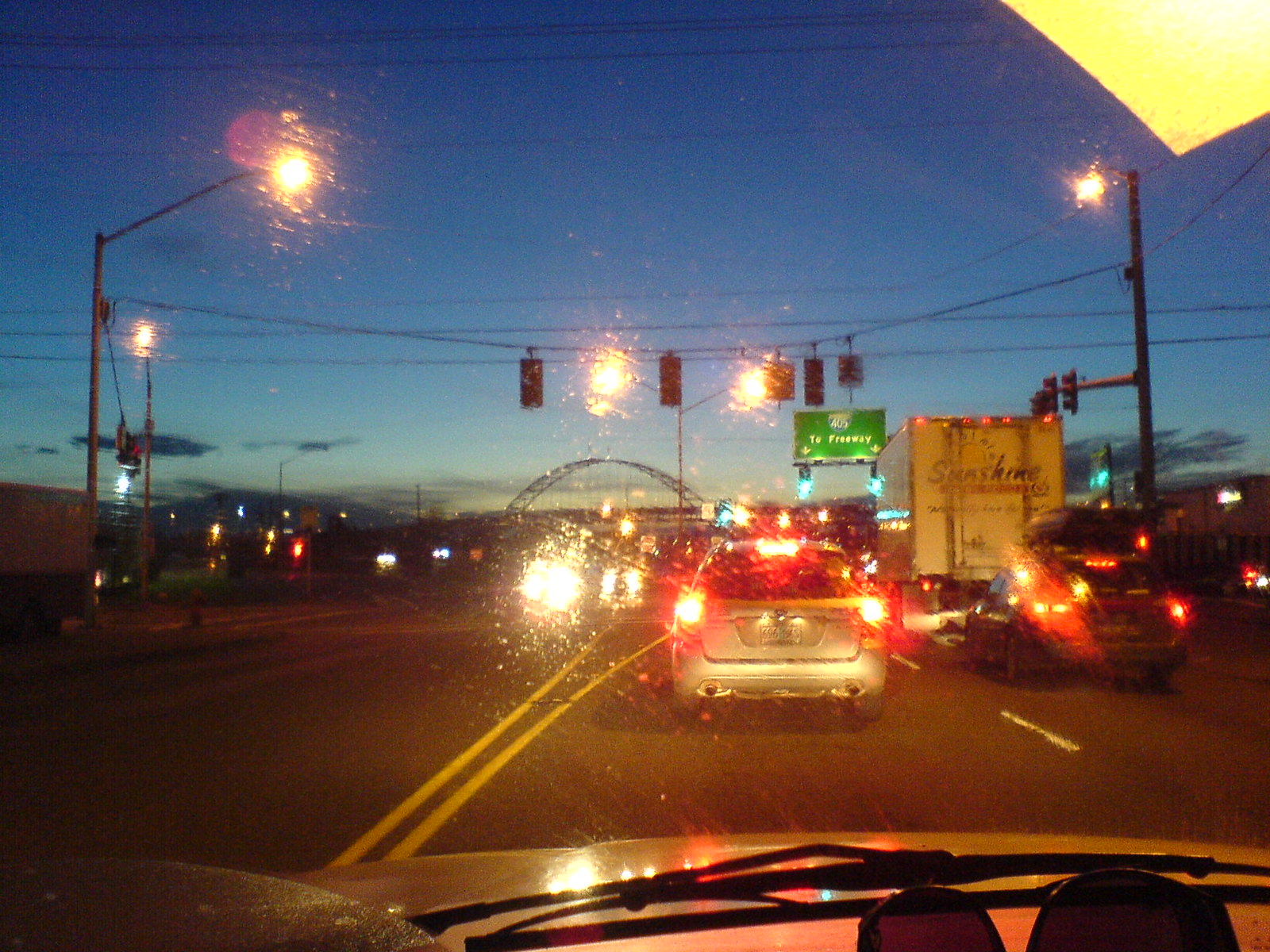This image, captured from inside a vehicle, possibly by a dash cam, depicts a scene at twilight or just after sunset, as evidenced by the dark blue hue of the sky. The view from the car window reveals a congested road filled with vehicles, indicated by the numerous taillights ahead. Streetlights have been turned on, casting a dim glow over the scene, while the headlights of oncoming traffic from the left illuminate the road in the distance. A green street sign, bearing the words "Two Freeway" and arrows pointing down, is also visible, directing traffic amidst the encroaching darkness. The atmosphere suggests a typical evening commute, marked by the interplay of artificial lights and the fading natural light.